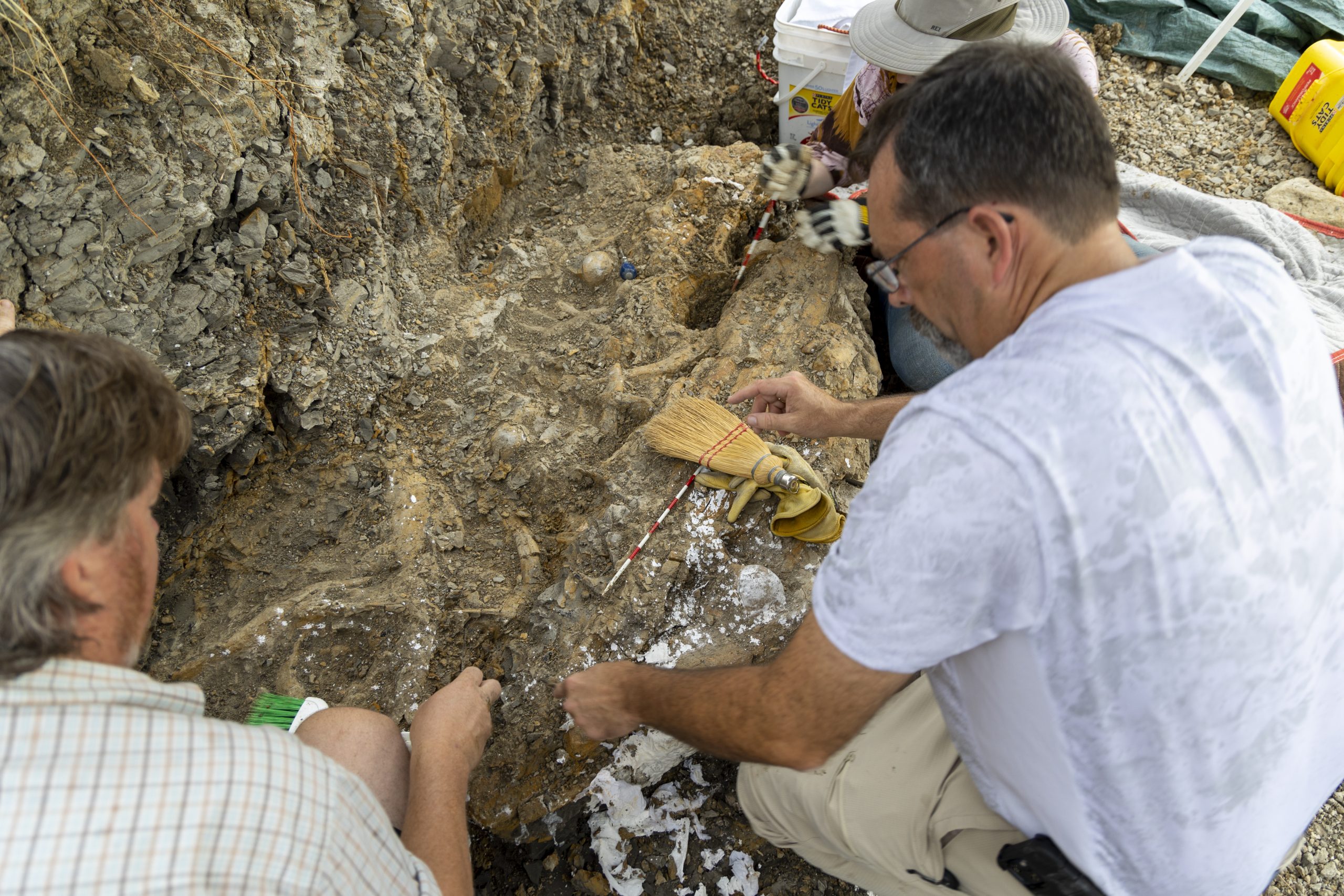In this image, three people are seen participating in an archaeological dig next to a large rock wall. They are working outdoors, close to a substantial rock that's connected to the wall, which has been intricately carved away to reveal some bones. These bones could belong to an ancient human, an animal, or even a dinosaur, though their exact nature is unclear. 

The trio is equipped with an array of tools, including small fine metal objects for picking and tiny brushes to clear away debris. Additional tools present include items that resemble red and white straws, a small tool akin to the top of a straw broom, and a chisel. They are also wearing gloves to protect their hands during the meticulous work. 

Nearby, there are buckets, one of which bears a Tidy Cats logo, suggesting repurposed containers likely holding excavation tools or collected samples. The scene depicts two men without hats and one individual wearing a hat, whose gender is indeterminate from the angle. The evidently intensive and detailed nature of their work underscores the careful process of unearthing and studying ancient remnants.